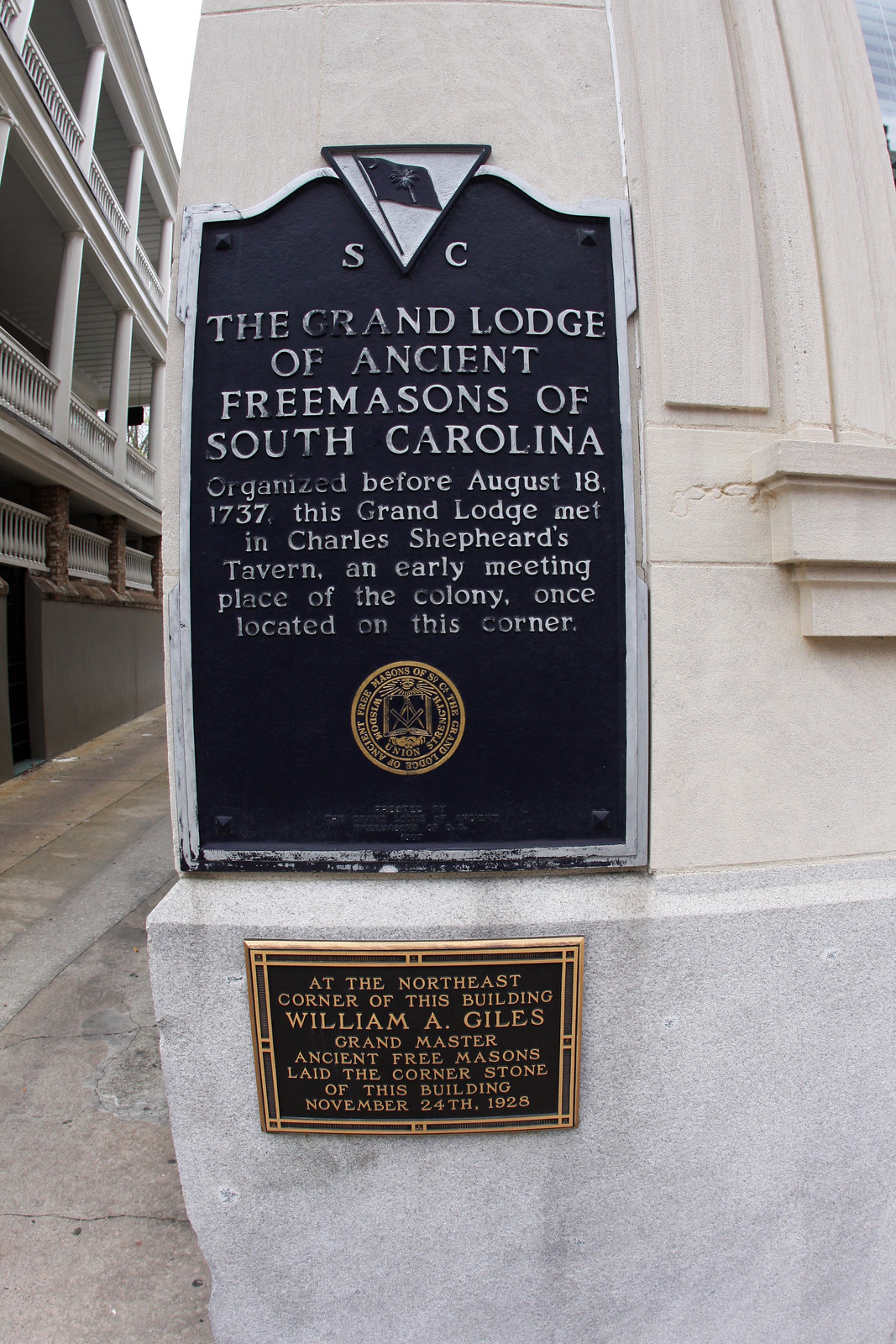The image showcases the exterior corner of a white building in daylight, with an alley on the left side and an adjacent building visible. Prominently displayed on this corner are two plaques. The top plaque, with a black background, features a blue flag and white text reading "SC" followed by "The Grand Lodge of Ancient Freemasons of South Carolina." It states that this Grand Lodge, organized before August 18, 1737, initially met in Charles Shepherd's Tavern, historically located at this very spot. Below the text is the seal of the Grand Lodge of Ancient Freemasons of South Carolina. The lower, smaller plaque has a brown and gold color scheme with gold lettering, noting that at the northeast corner of this building, William A. Giles, Grand Master of Ancient Freemasons, laid the cornerstone on November 24, 1928.